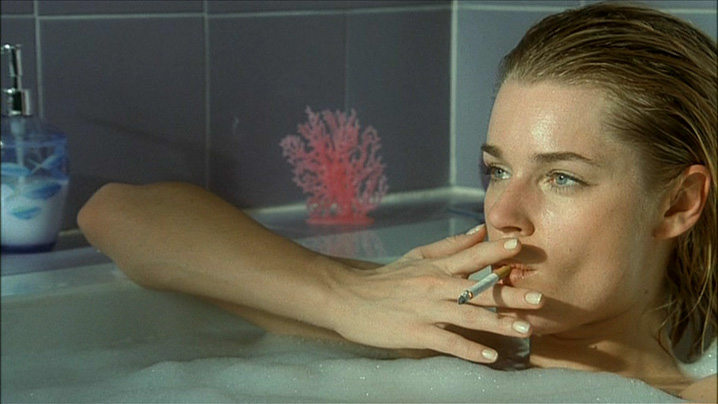The photograph captures a young woman in her early 20s submerged in a bubble-filled bathtub, with visible portions from her shoulders upwards. Reclined in the tub, she has wet, slicked-back hair of blondish-brown color. Her right arm is propped on the side of the tub, and her well-manicured white fingernails are poised to grasp a lit cigarette that rests between her lips, the orange tip pointing inward. She gazes thoughtfully to the left of the image. The background showcases purplish-blue tiles and two decorative elements: a blue fish-covered soap dispenser on her left and a pink coral ornament above her arm on the tub's edge. The photograph, characterized by photographic realism, is in a landscape orientation.